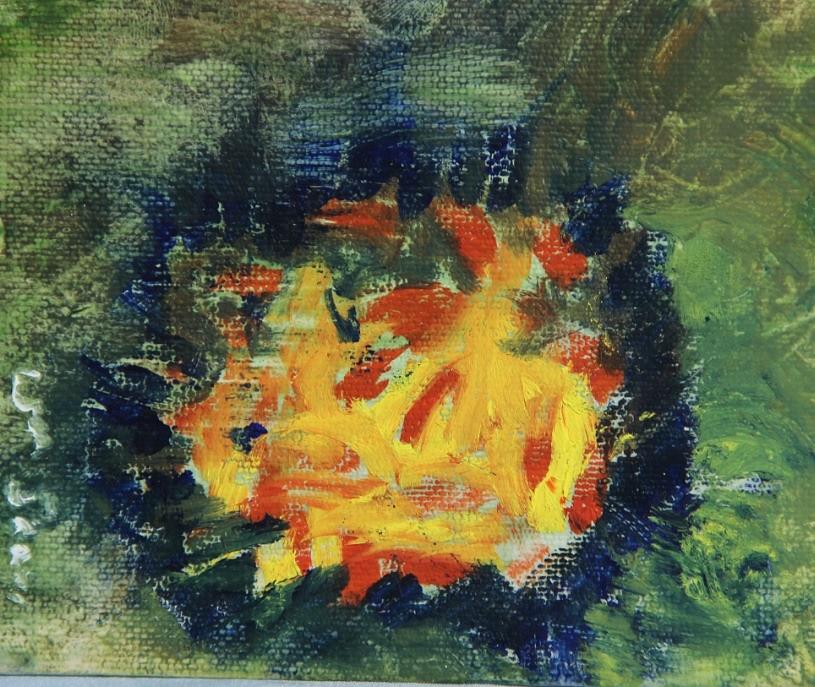This oil-on-canvas painting, signed in white on the left-hand side though the artist's signature is illegible, features a compelling abstract composition with dynamic brushwork and vivid colors. The border of the painting is characterized by broad, swirling strokes of green and tan hues, reminiscent of camouflage patterns, possibly suggesting a forest landscape. In the middle section, single, abrupt upward brush strokes of dark blue pigment create a central circular form. Within this circle, fiery red, orange, and yellow strokes burst forth in multiple directions, reminiscent of a campfire's flames. The contrasting colors and varied brushwork create a sense of chaotic energy while drawing the eye towards the vibrant center. The overall impression is that of a roaring campfire surrounded by bluish-black elements, akin to stones, set against a verdant backdrop, possibly hinting at grass or trees. This busy, multi-layered painting utilizes the contrast between the structured borders and the explosive center to evoke a powerful visual and emotional experience. The true meaning of the piece remains open to interpretation.